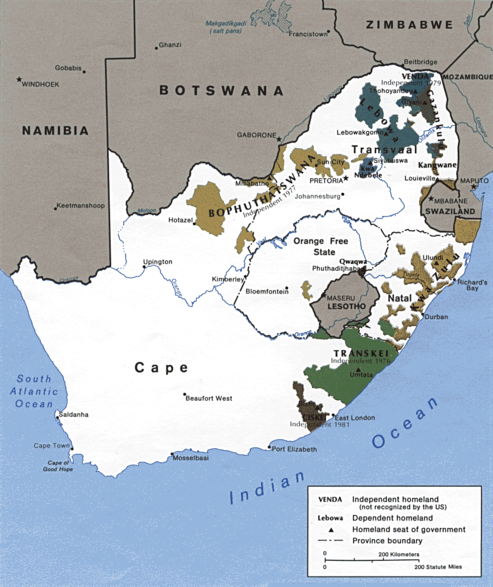The image is a detailed screenshot of a map resembling South Africa, though notably, South Africa has been renamed "Cape." To the left and bottom right of "Cape," the South Atlantic Ocean and Indian Ocean are depicted in blue, while the neighboring countries Namibia, Botswana, Zimbabwe, Mozambique, and Eswatini (formerly Swaziland) are illustrated in black and gray hues. Additionally, this map showcases a significant reconfiguration where numerous smaller regions have been delineated within what traditionally constitutes South Africa. These regions are marked in various colors: an unidentified brown area in the bottom right, a green region labeled "Transkei," and further subdivisions in the upper northeast labeled "Bala," "Venda," and "Butsa." It seems that these names might represent traditional tribal lands or proposed administrative regions. The portrayal suggests a hypothetical or alternative geopolitical arrangement of the area, possibly indicating how someone believes the territory should be divided.